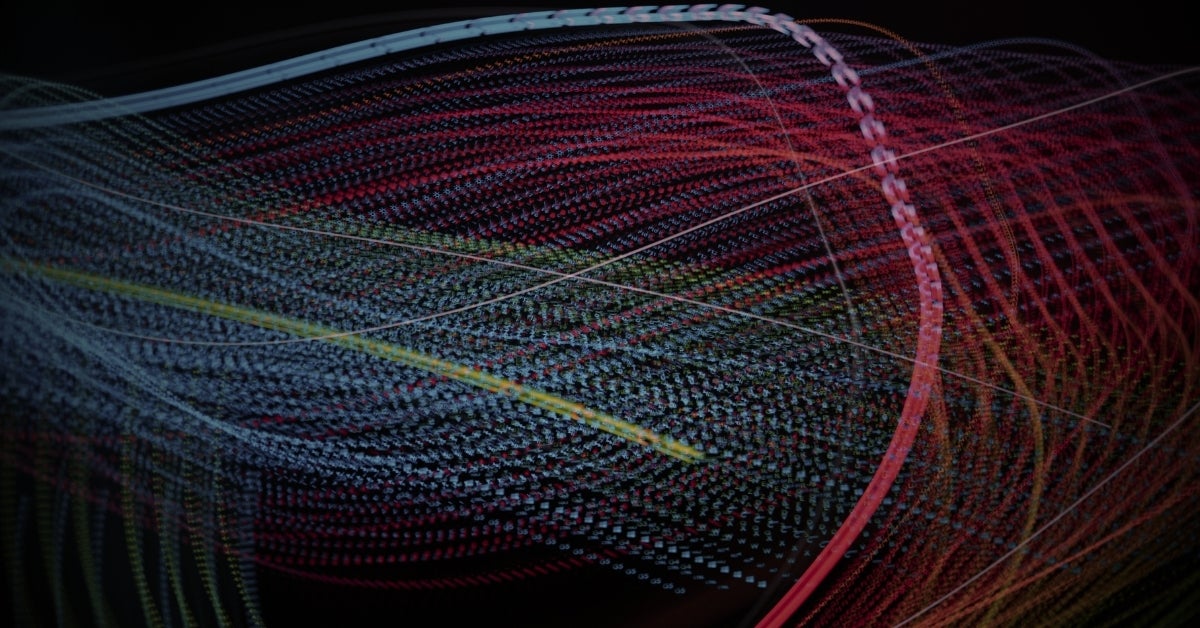This horizontally rectangular, digitally created abstract art piece features a black background with an intricate web of colorful lines. The composition is primarily dominated by thicker lines that wind across the image. Starting from the upper left corner, a thick, grayish line curves and gradually transforms into red as it exits at the bottom edge. This main line intersects with another smaller, thick red line. Thin red and gray lines subtly extend from this intersection toward the edges of the piece, creating a layered look.

Additionally, thicker blue lines weave into the pattern, transitioning from red at the bottom, looping upward and turning blue as they move to the left. Complementing this, thin blue lines crisscross horizontally across the composition, providing a sense of fluid movement. A distinct, yellow line slices across the image's middle but stops short of the edges, sitting above some underlying gray lines. A green line also stands out near the center, adding to the colorful complexity of the design. The overall effect of these interlacing lines is reminiscent of rope, creating a visually compelling and dynamic artwork, possibly reminiscent of a screensaver or desktop background.